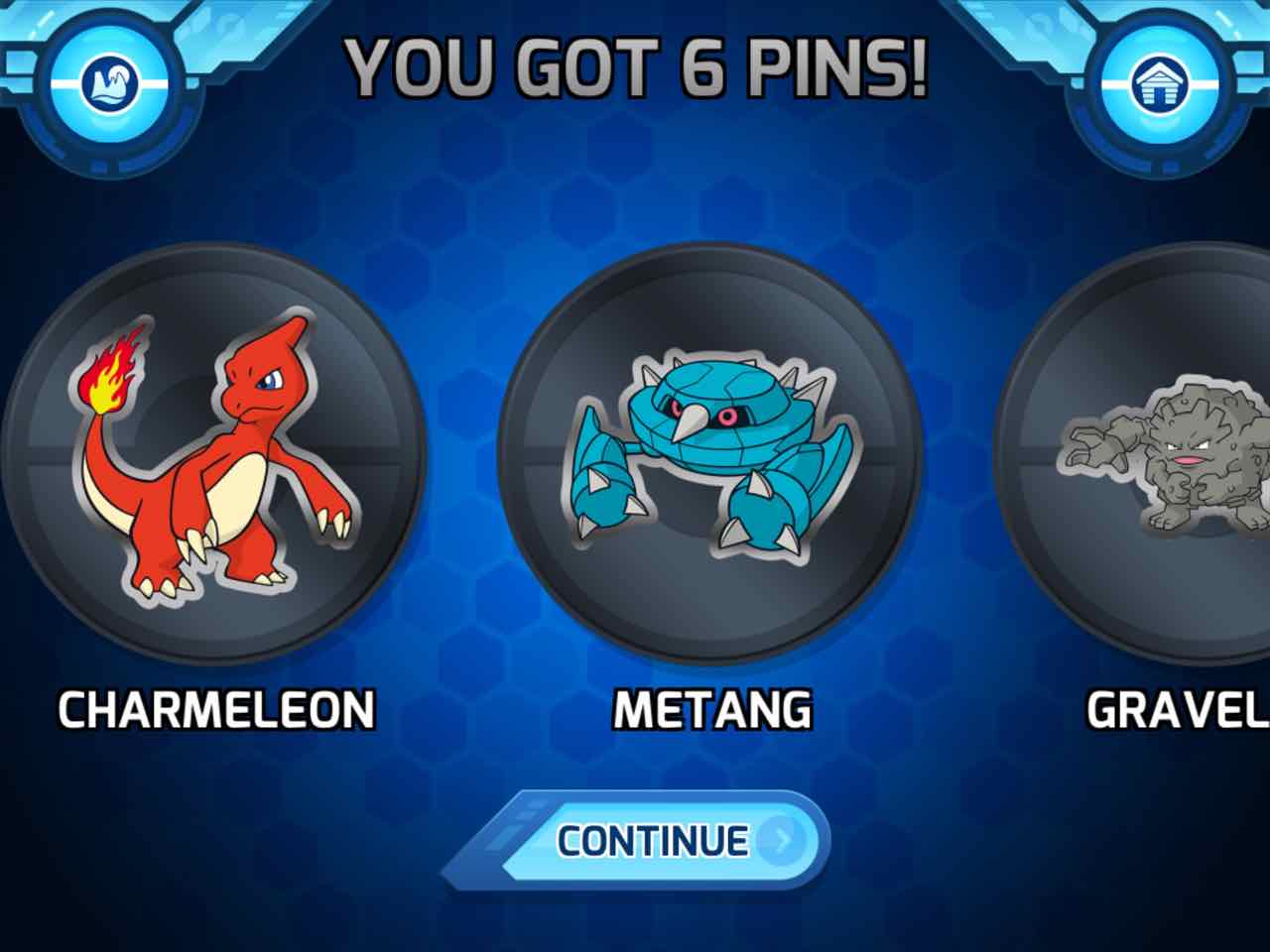The screenshot showcases a video game scene with a predominantly blue background featuring a hexagonal pattern in varying shades of blue, from light to dark, which gradually fade into black at the corners. At the top, the text "You got six pins" is displayed in gray letters. Below this, three black circles are aligned horizontally. The left circle contains an image of a red dinosaur-like creature with a fiery tail, identified as Charmeleon. The middle circle presents a blue creature with a sharp nose, red eyes, and sharp claws on its arms, named Metang. The right circle features a gray, dust-like rock creature with white eyes and a pink mouth, named Graveler. Additionally, a blue "Continue" button is visible at the bottom of the screen.